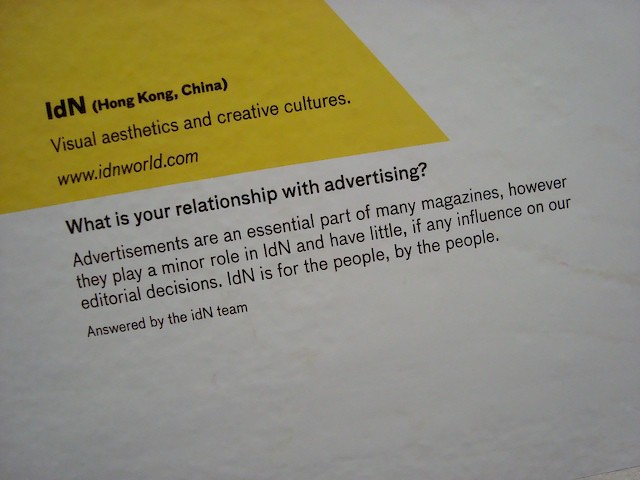This photograph features a piece of promotional material for the public relations company, IDN. The layout is predominantly white with a section of yellow shading in the upper left corner. The bolded black text within this yellow section reads "IDN (Hong Kong, China)," with "IDN" in larger font and the "IN" of IDN in lowercase. Below this header, it states "Visual Aesthetics and Creative Cultures" alongside the company’s website, "www.idnworld.com."

The main body of the text follows, starting with the bold black question, "What is your relationship with advertising?" This is followed by a paragraph in regular black font that elaborates on advertising’s role in magazines, stating that while advertisements are essential in many publications, they play a minor role in IDN and do not influence the magazine's editorial decisions. The text reinforces IDN's commitment to being "for the people, by the people." The passage concludes with the note, "Answered by the IDN team." The structure, color usage, and textual content combine to create a detailed and cohesive promotional flyer for IDN’s services and philosophy.